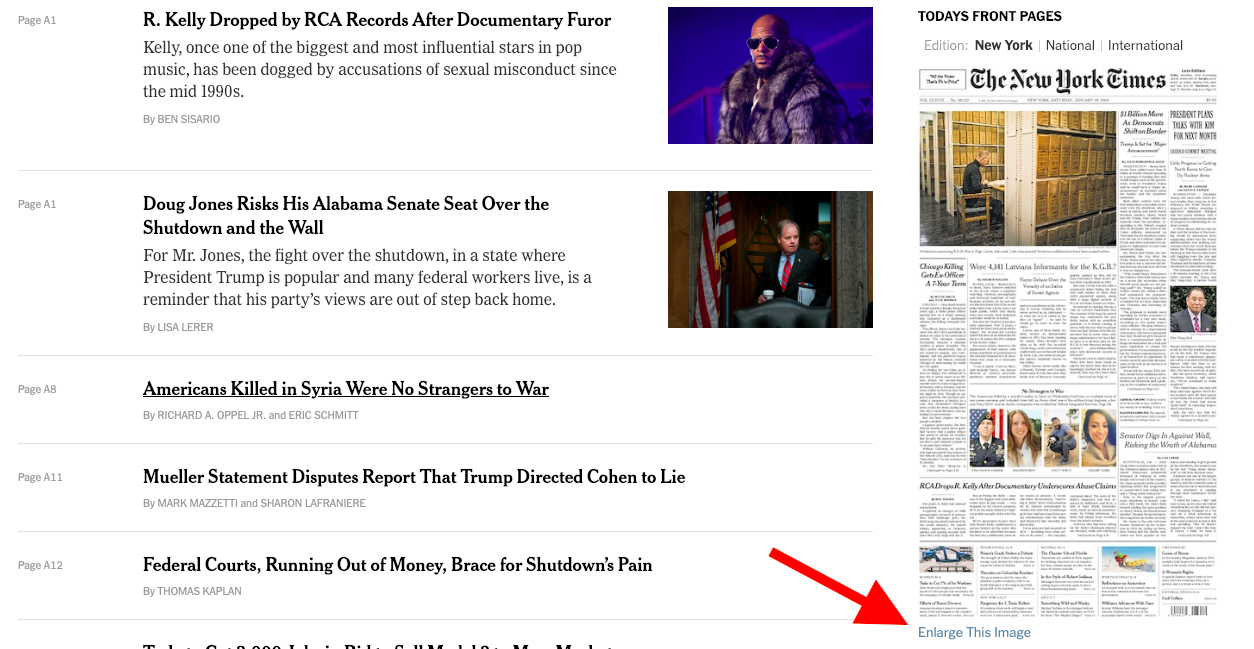The image depicts a website showcasing the New York Times, with a split view of their front page and a list of highlighted articles. On the right side, the front page of the New York Times is prominently displayed, labeled "Today's Front Pages," followed by the edition types: New York (bold), National, and International. 

On the left, there is a detailed list of article links, each marked by their respective page numbers. The first entry is for Page A1: "R. Kelly Dropped by RCA Records After Documentary Furor," accompanied by a brief description in smaller gray font, detailing that Kelly, once a significant figure in pop music, has faced accusations of sexual misconduct since the mid-1990s, written by Ben Cesario. 

The second entry, also on Page A1, is "Doug Jones Risks His Alabama Senate Seat Over the Shutdown and the Wall," highlighting the Senate fight in a Trump-supporting state, authored by Lisa Lerer. 

Following that, on Page A8, is the article "Americans Killed in Syria Were No Strangers to War," marked by an underline and no synopsis, penned by Richard A. Oppel Jr. and Eric Schmitt. 

Page A11 focuses on "Mueller's Statement Disputes Report That Trump Directed Cohen to Lie," authored by Mark Mazzetti and Sharon LaFraniere. 

Lastly, Page A12 covers "Federal Courts Running Out of Money Brace for Shutdown's Pain" by Thomas Kaplan.

Beneath the front page image of the New York Times, a prominent red arrow points towards the blue text "Enlarge This Image."